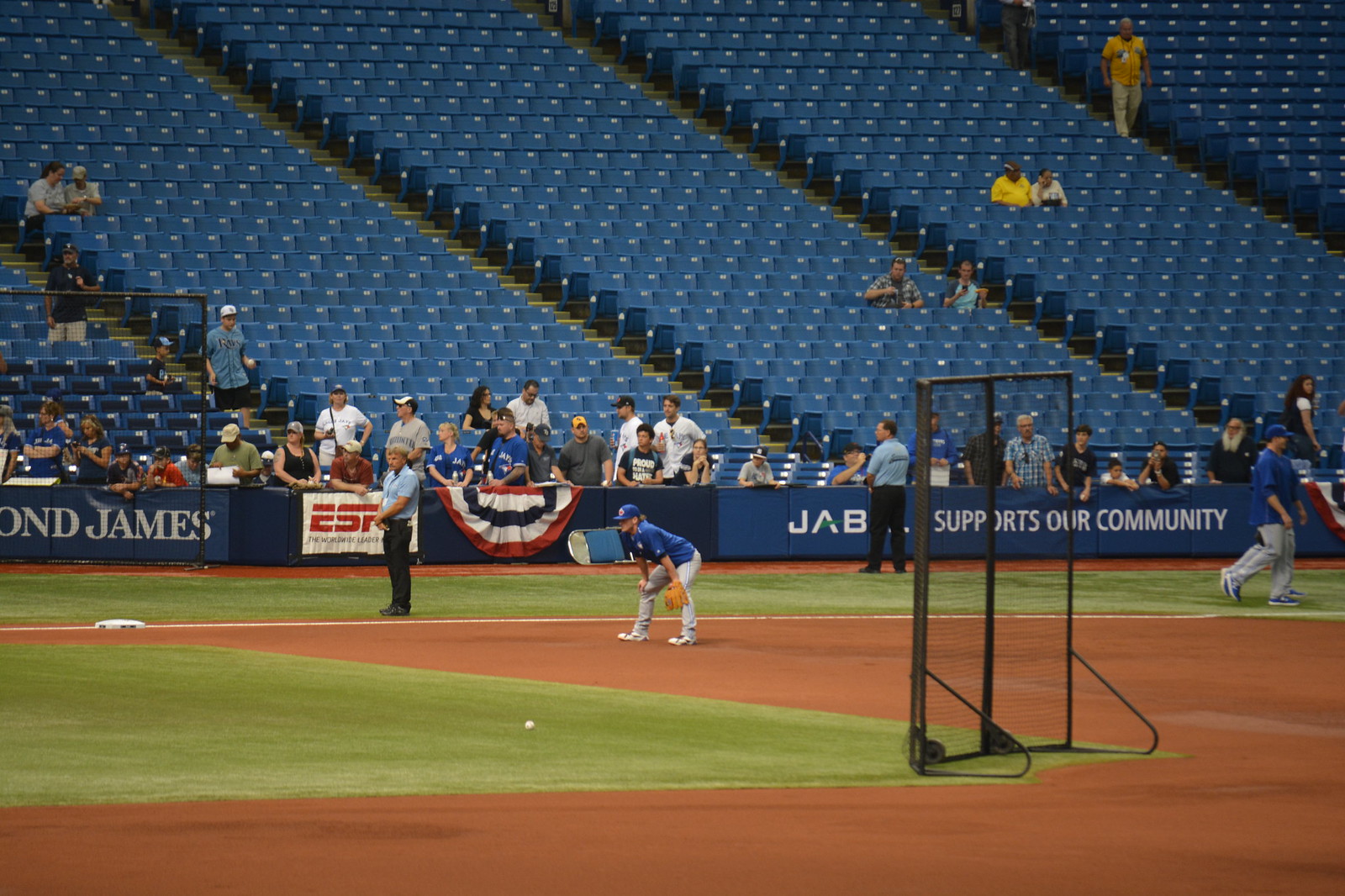The image captures an outdoor baseball game scene with a detailed view of a baseball diamond in the forefront. The field is characterized by green grassy areas and brown muddy patches, indicating the distinct zones of play. On the left-hand side of the image, one of the bases is visible. A player, dressed in long gray pants, a blue short-sleeved shirt, and a blue baseball cap, is crouching with a mitt in hand, seemingly in a defensive stance. An umpire is standing nearby, also on the left-hand side of the field. Another player can be seen on the right-hand side, walking sideways, adding to the dynamic nature of the scene. Behind them, there is a sign displaying various sponsors, including JAB and ESPN, with messages supporting the community. The background reveals an almost empty stadium with multiple levels of blue seats, suggesting that the game might be in its early stages or during a practice session. The overall scene conveys a tone of preparation and anticipation, with a few spectators sparsely scattered in the stands and security personnel standing around.